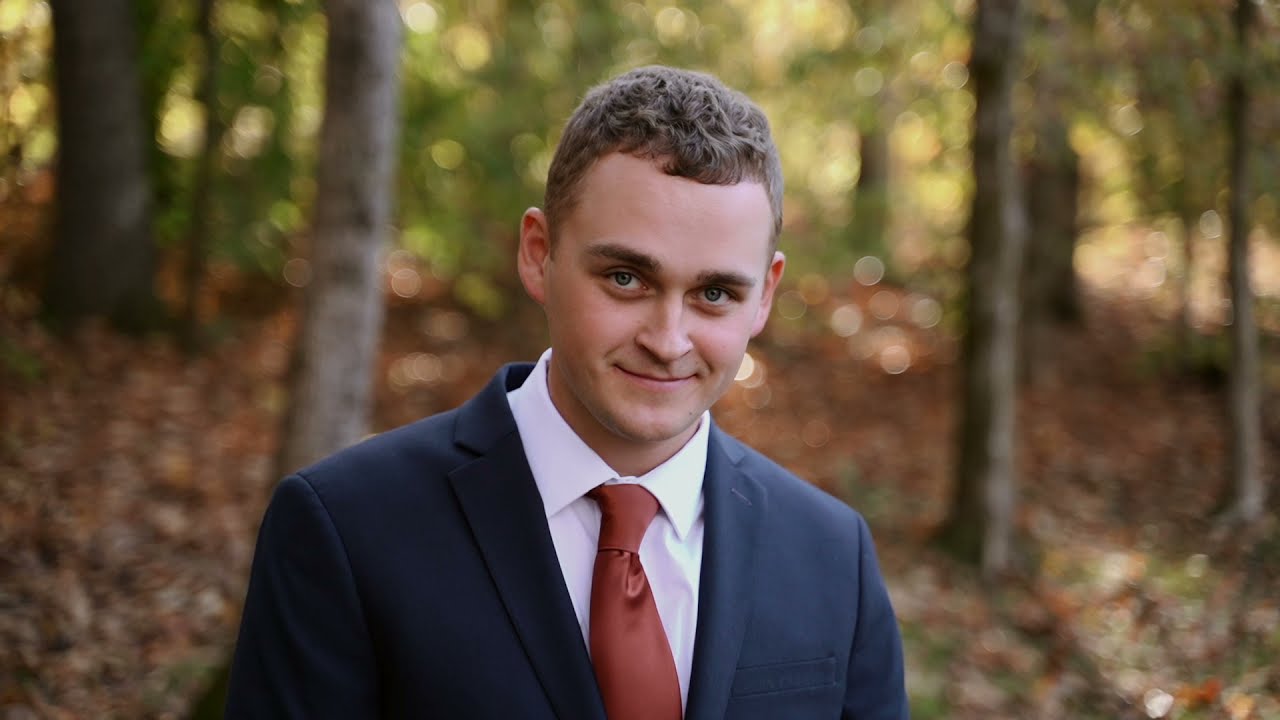The image depicts a clean-shaven young man in his late 20s with blue eyes and short, light brown, slightly wavy hair. He has a smooth face with blond eyebrows and minimal sideburns. The man is donning a navy blue suit paired with a white button-up shirt and an orange-burgundy tie. He appears to be smiling with a closed mouth as he gazes into the camera. The background is unfocused, showcasing a blurry scene of a fall forest with gray tree trunks and scattered leaves on the ground, giving the image a professional, bokeh effect. This could possibly be a graduation picture, capturing a serene and celebratory outdoor setting.